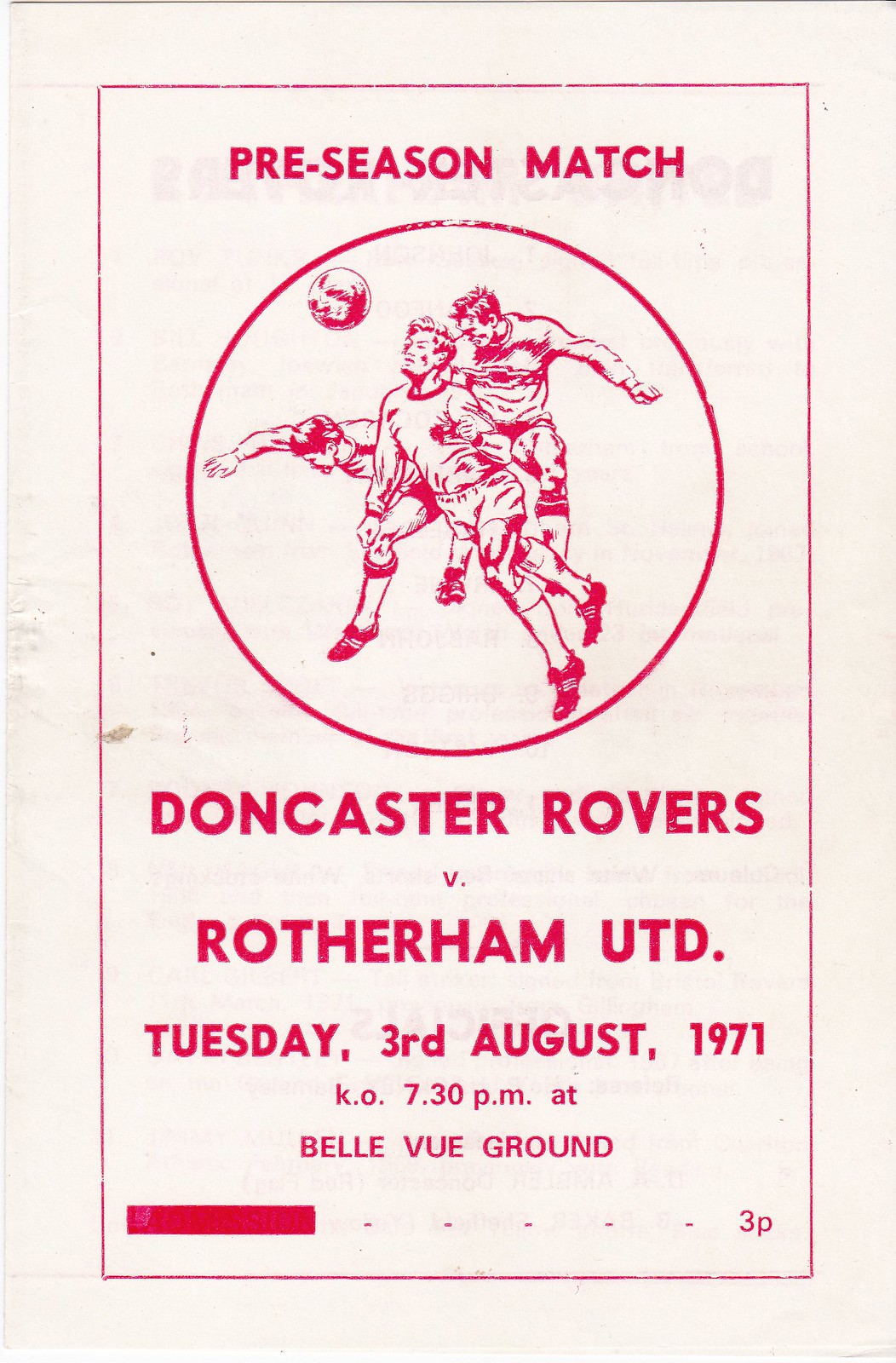An advertisement for a pre-season soccer match is set against an off-white background framed by a red square. At the top, in bold, capitalized red letters, it prominently announces "PRE-SEASON MATCH." Below this, a red circle contains an illustration of three soccer players actively engaged in pursuing a soccer ball. The player on the left is leaning forward with an outstretched hand, the player in the center balances on one toe with a focused header towards the ball, and the player in the back, identifiable by a shirt bearing a Chevy emblem, extends an arm to the side. Beneath the circle, red block text details the event: "Doncaster Rovers vs. Rotherham UTD, Tuesday, 3rd August 1971, K.O. 7.30 p.m. at Bellevue Ground." At the bottom, a red bar on the left side ends abruptly with five dots trailing off, followed by "3P" indicating the price or page.